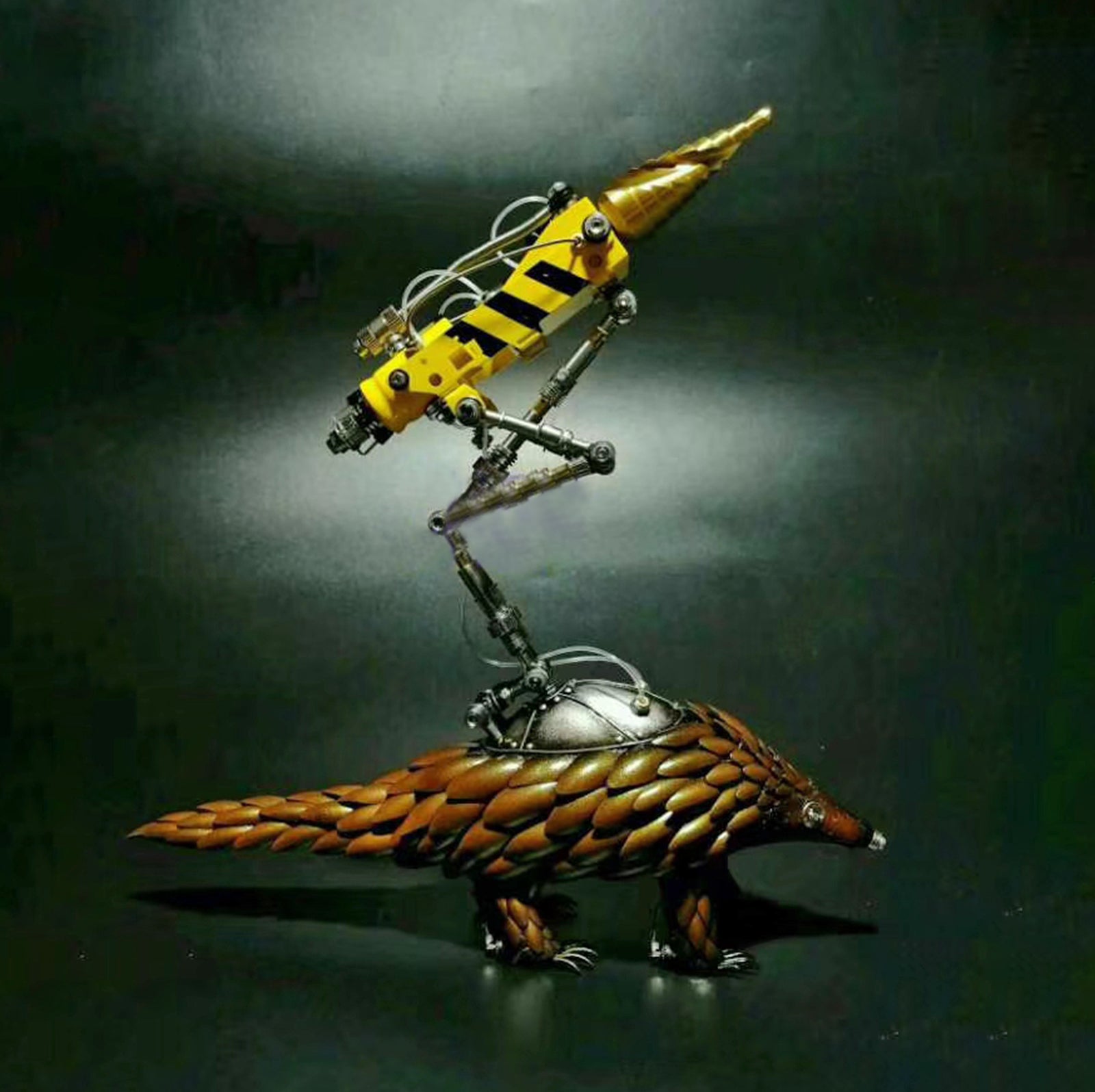This detailed image features a computer-generated portrayal of a peculiar figurine, set against a grayish-green background with soft, whitish lighting that gives it a vintage feel. At the base is an animal resembling a cross between a platypus and an armadillo, characterized by brown, armor-like, scaly skin. Its body includes distinct features such as silver claws on its feet, a cone-shaped face with a visible right eye, and it appears to be crafted from a shiny, metallic material.

Mounted on top of the animal is a complex robotic apparatus, positioned on a pivot that functions similarly to a tripod. This apparatus has a silver base and legs. The robot component is colorfully detailed with a red and black body, intricate wiring, and a yellow cylindrical segment adorned with black stripes. Prominently extending from the front of this robot is a projectile-like object resembling a missile or weapon, with a conical shape distinguished by bands of gold and a sharp point, suggesting the capability for drilling or penetration. The combination of organic and mechanical elements in this figure creates a unique, futuristic aesthetic.